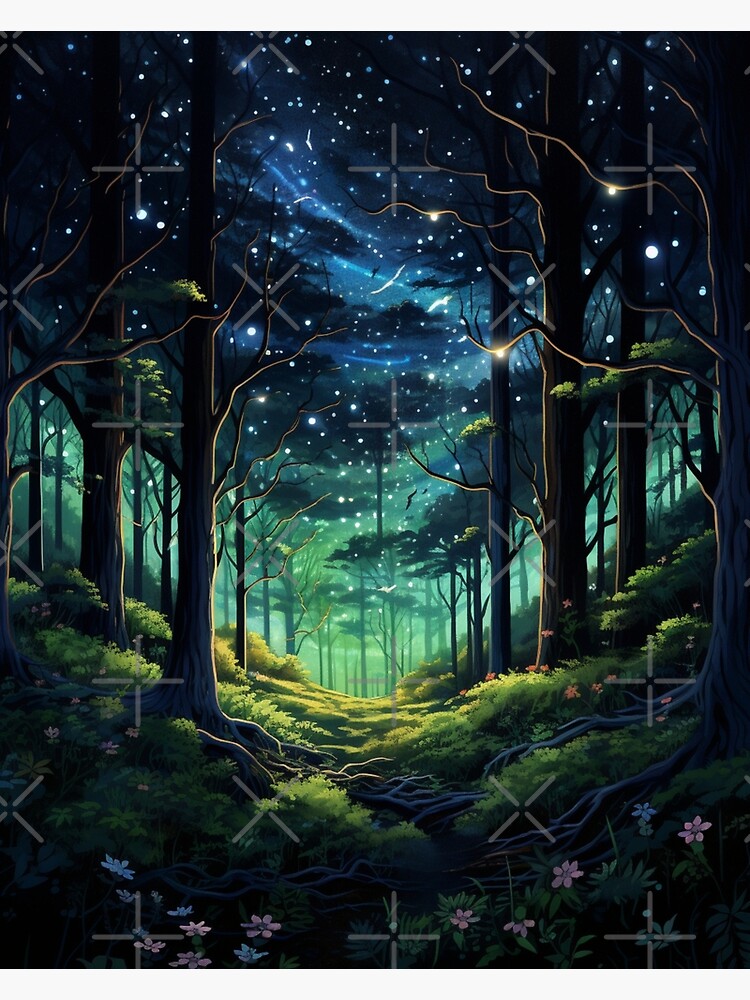The image depicts a stunning nighttime digital art scene of a dense forest, where tall, mostly bare trees line the left and right perimeters, creating a mirrored, U-shaped valley that descends into the center. The ground is adorned with a mix of green grass, shrubs, and vividly colored flowers, with distinct petals in hues of blue and red or pink. The night sky above transitions from black at the top to a bluish tint, punctuated by numerous stars and lights that resemble perfect white circles, with some areas displaying a greenish-turquoise luminosity. Faint crosses or X marks are scattered across the sky, adding an abstract touch without detracting from the overall beauty. The interplay of darkness and the night sky's illumination cast a mystical, almost otherworldly atmosphere over the well-lit scene, emphasizing the enchanting blend of natural and digital artistry.